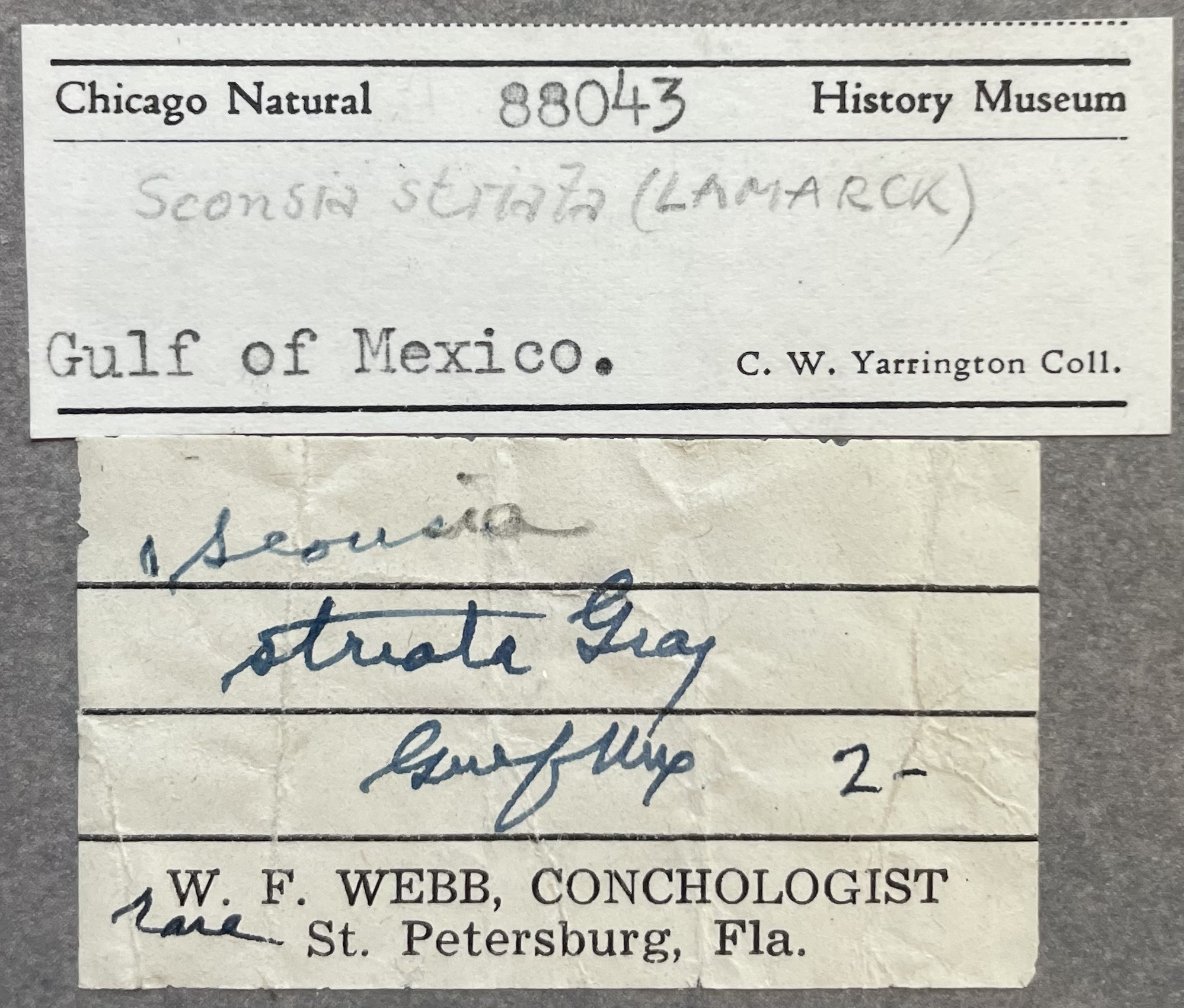This image contains two aged, slightly wrinkled labels placed against a gray background. The top label is white and features black typed lettering. Across the top, it reads "Chicago Natural" followed by the numbers "88043," and "History Museum." Beneath this in pencil, handwritten text spells out "Scanasia Striata (Lamarck)" followed by "Gulf of Mexico." To the right, it states "C.W. Yarrington, C-O-L-L." A prominent horizontal black line runs through part of this label. The second label, positioned below the first, is off-white and also shows signs of age. It repeats the name "Scanasia Striata" in handwritten ink, with additional pen notations. At the bottom of this label, it reads "W.F. Webb, Conchologist, St. Petersburg, Florida" in print. Both labels provide a historical record associated with specimens and collectors, marked by meticulous though somewhat faded details.